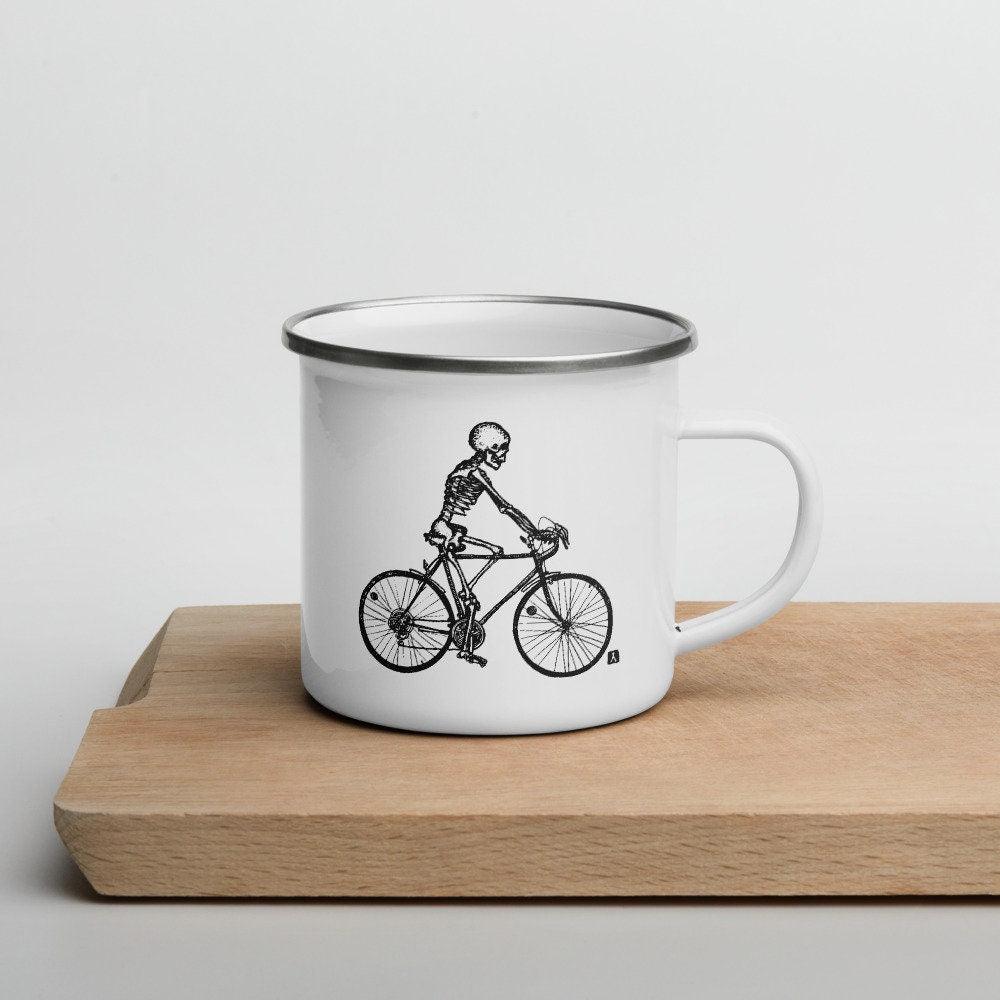The image displays a light-colored wooden slab serving as a platform, set against a gradient background that transitions from white at the top to light gray at the bottom. Positioned atop the slab is a white enamel mug with a large, white handle and a distinctive black rim around its top. The mug features an artistic black outline of a skeleton riding a bicycle, with one leg positioned to pedal and detailed elements like visible ribs and reflector markings on each tire. In the bottom right corner of the skeleton artwork, a small black and white logo is present. The overall composition includes only these two primary objects—the mug and the wooden slab.